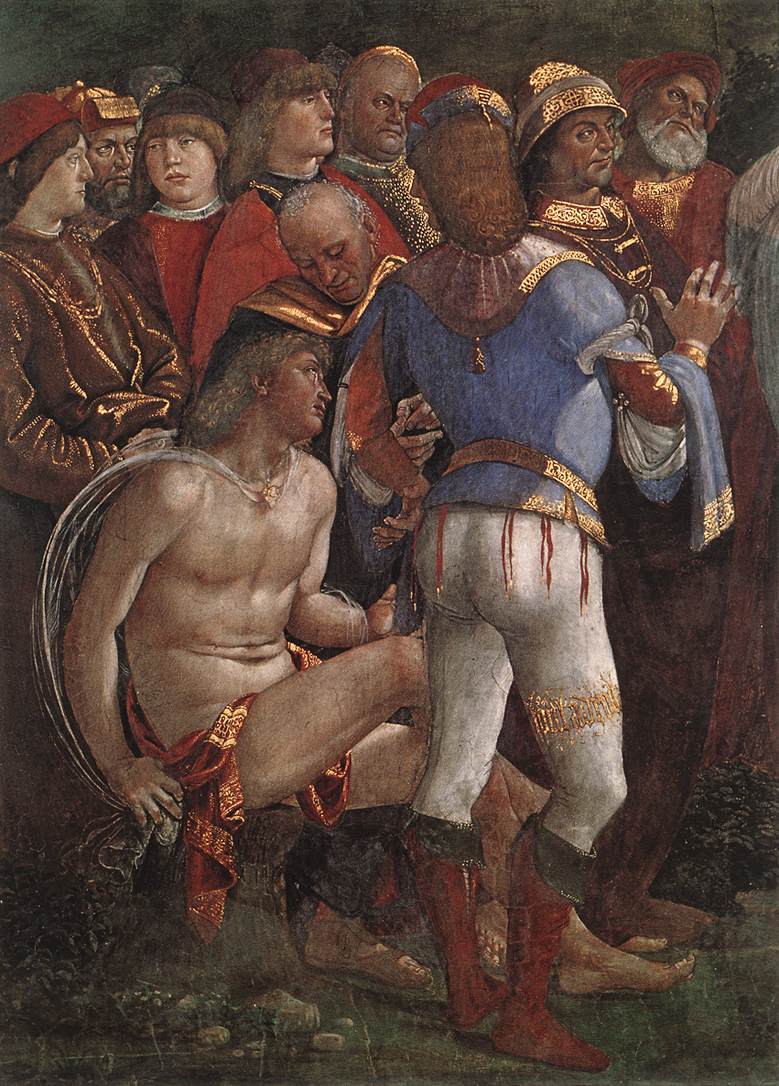This detailed painting, rendered in what appears to be aged and cracked oil paint, showcases a dramatic and solemn scene set against a dark sky. The central figure is a nearly naked man with long hair, seated and covering his modesty with a red cloth. His muscular physique and the cape tied around his neck suggest a warrior-like presence. He is surrounded by an assembly of people dressed in luxurious, colorful, and richly ornamented clothing, indicative of upper-class status or royalty. Their attire includes ornate robes with gold embellishments, headgear, nice trousers, and boots, resembling priests or military figures with detailed uniforms. One notable man, situated to the right, stands out in a jester-like blue and white spandex outfit, possibly performing crowd control. This figure adds a unique element to the scene, contrasting sharply with the otherwise solemn and regal attire of the crowd. Among the onlookers, an older man directs a gaze filled with disdain or contemplation towards the seated figure, while another man, whose back is towards the viewer, raises his hand as if making a point. The crowd appears to be lined up, all heading in one direction, except for a single individual smirking at the peculiar scene. This painting captures a complex tableau filled with contrasting emotions and intriguing character interactions.